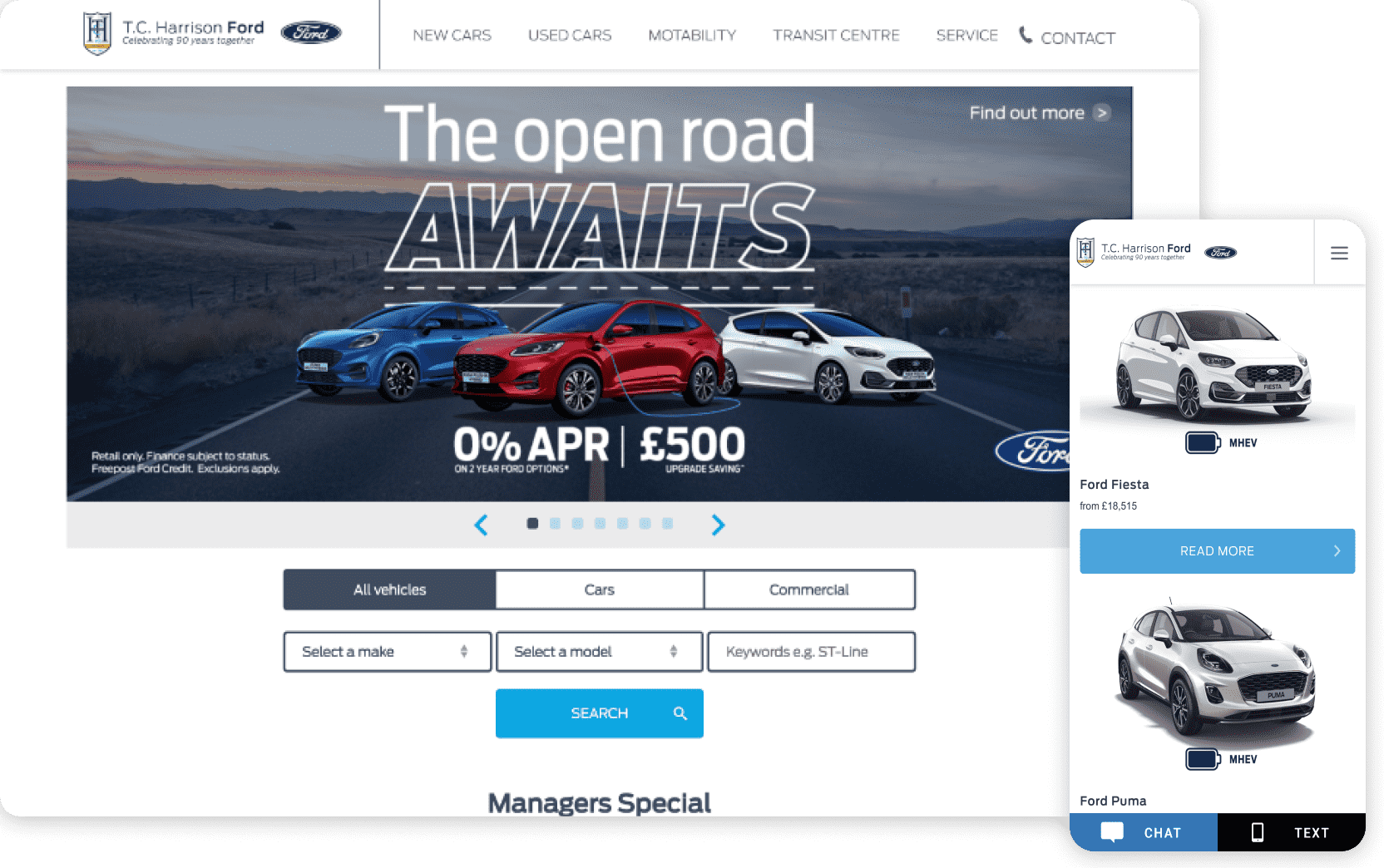This website showcases T.C. Harrison Ford, prominently featuring a SHIELD logo on the left-hand side along with the company's name, followed by the iconic Ford logo. Below the name, a message reads, "Celebrating 90 Years Together." On the right-hand side, a navigation bar includes sections for New Cars, Used Cars, Motability, Transit Center, Service, and Contact. The central image displays three vehicles: a blue car, a red car, and a white car, positioned on a road with the caption "The Open Road Awaits" above them. The background highlights a scenic landscape with mountains and prairies flanking the road. In the upper right corner of this image, "Find Out More" with a right-pointing arrow is written in white. Below the cars, the text reads "0% APR / £500, with the Ford logo seen on the bottom right-hand side. Additionally, two white cars - a Ford Fiesta and a Ford Puma - are displayed in white boxes on the right-hand side, each accompanied by a "Read More" link. Beneath the main image, boxes are labeled All Vehicles, Cars, Commercial. Further down, options for selecting a Make, Model, and adding Keywords are provided, alongside a Search button and a section titled "Manager Special."